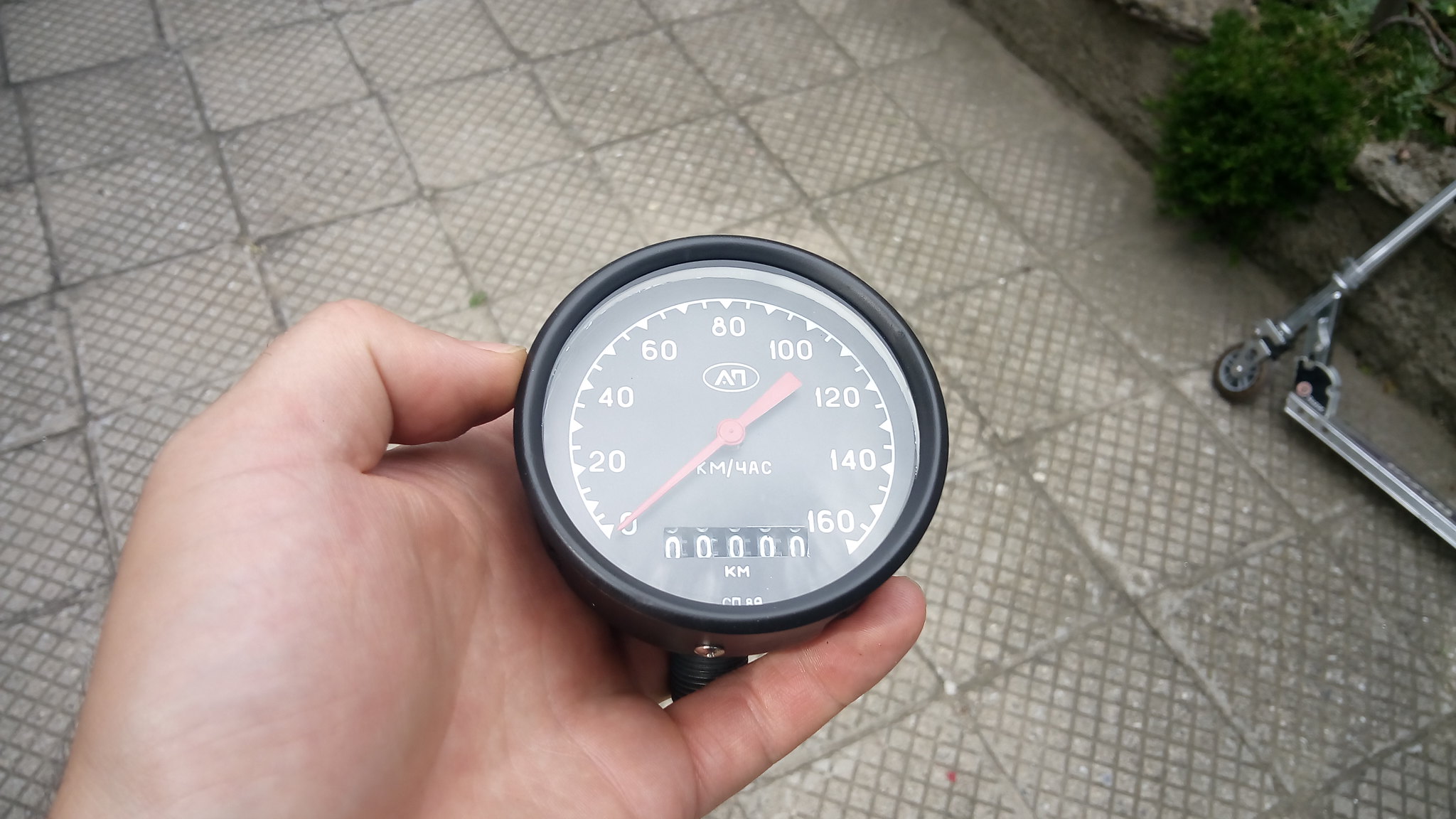In this photograph, a light-skinned hand, possibly of Caucasian or Asian descent, is holding a gauge with a black plastic casing and a glass front. The dial face ranges from 0 to 160, marked by white increments on a dark background. A prominent red pointer indicates the current reading. Below the dial, a rolling counter is visible, all set to '000000 km', suggesting the gauge may be new or reset. This device could be a speedometer for a motorcycle or a dirt bike. To the right of the image, a scooter leans against a wall draped with a lush, overhanging shrub. The ground beneath is paved with crosshatched stones, adding texture to the setting.